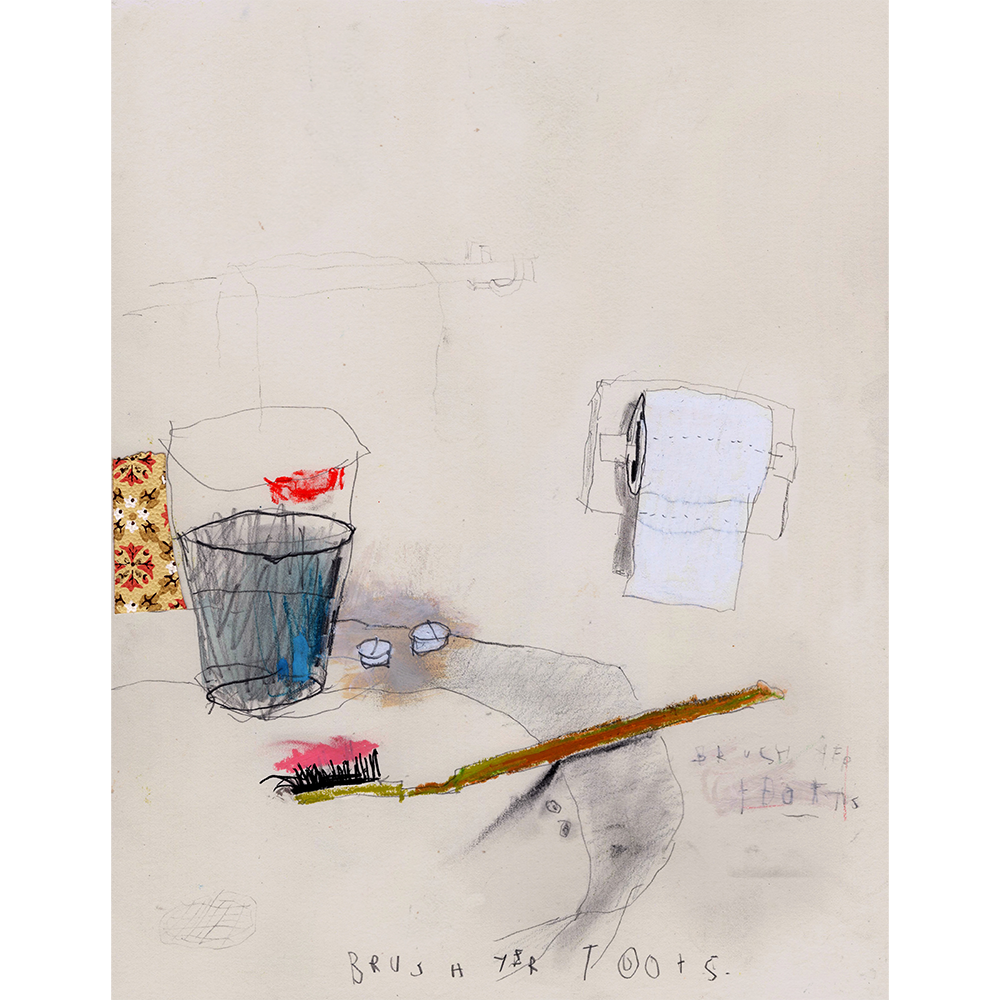This illustration depicts a collection of bathroom items set against a beige background. On the left side, about halfway down the image, there is a small section of wallpaper featuring a beige background adorned with brown and red flowers. Below this decorative strip is what appears to be a sink or table. Resting on this surface is a container resembling a trash can; it is gray with a rounded top. Above this container, there are outline sketches hinting at a taller trash can, marked with a small pink spot and a touch of blue inside the can.

Adjacent to this container, there are two small, flat, white circular objects that resemble buttons. Positioned near these objects is a brown toothbrush with black bristles, which has a smear of pink toothpaste on it. This toothbrush is lying flat on the surface of the sink or table.

The edge of the sink or table is gray, and beneath this edge, there is a text that reads "brush your toots." Although there is additional writing located under the handle of the toothbrush, it appears blurry and is illegible.

Above this area, mounted on the wall, is a toilet paper holder. The holder itself is beige, while the toilet paper it contains is white.